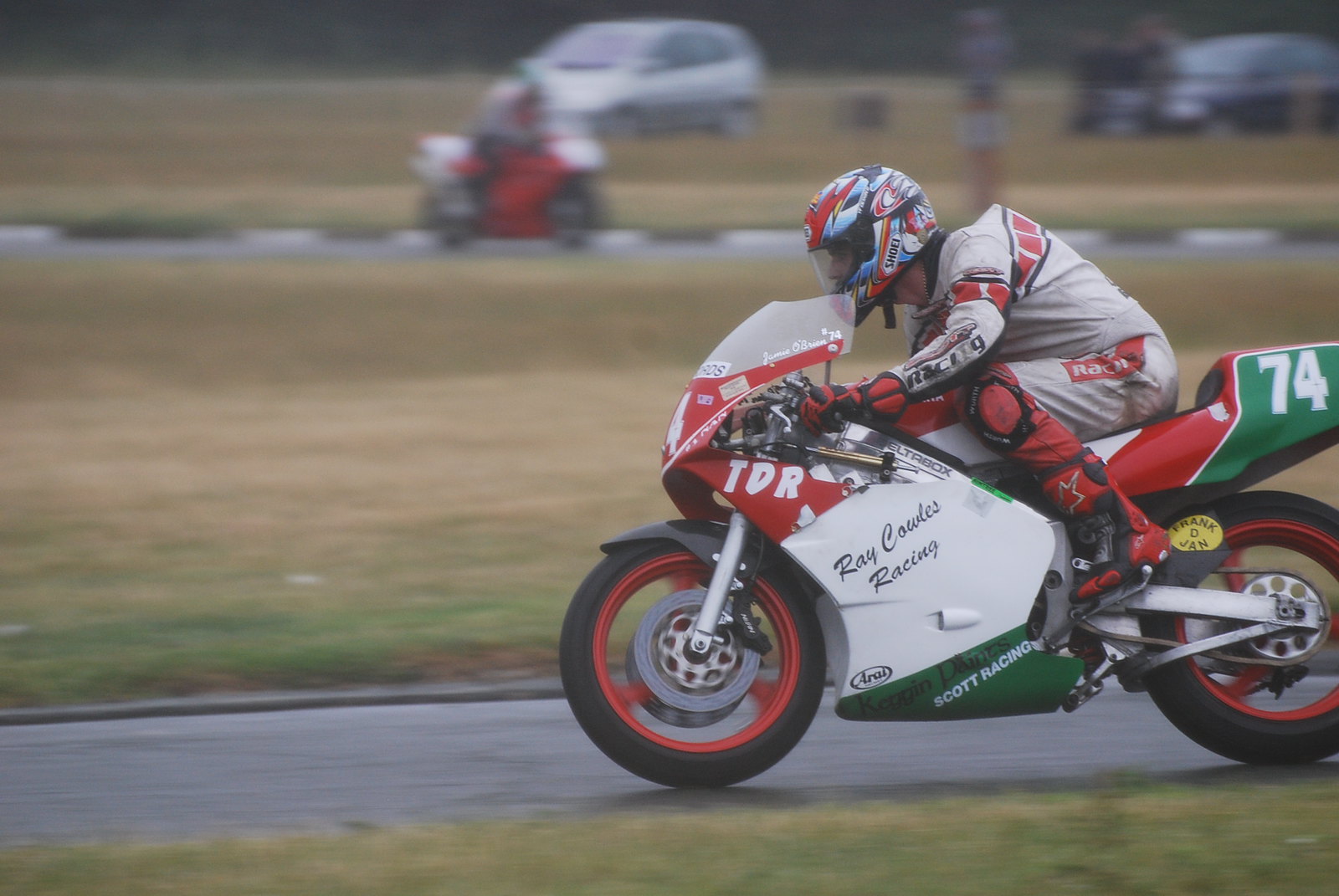This is a dynamic photograph captured at a motorcycle racing track, vividly portraying a rider and his motorcycle. Dominating the foreground, the rider is clad in a white racing suit adorned with red accents and the word "Racing" on his front arm. His helmet, which features an elaborate design primarily in blue with notes of red and black, has a clear visor at the front. His red and black gloves and boots complement the outfit. The motorcycle he rides is striking, with a red front and a white body, transitioning to a green rear section with the number 74 displayed prominently. The rims are also red. The text "Ray Cowles Racing" is visible on the white side panel of the motorcycle. The image exudes a sense of speed, as the slightly blurred background and foreground suggest rapid motion. Off to the right but moving left, the motorcycle is not perfectly centered, enhancing the feeling of dynamic movement. In the distant background, another red motorcycle appears, although it is quite blurry, along with some cars visible near a parking area, further emphasizing the sharp focus on the main subject.